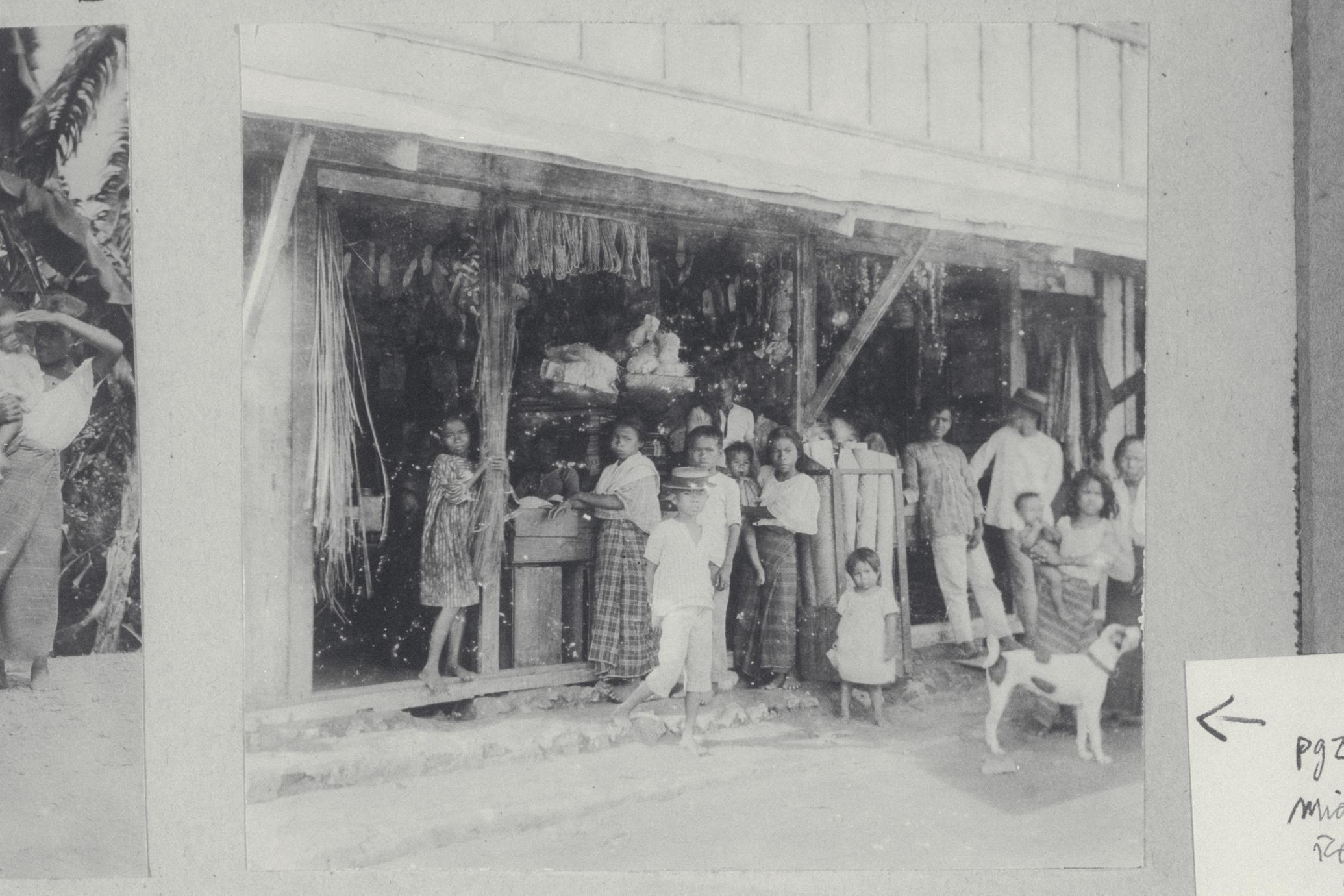This is a detailed black and white photograph capturing a group of African Americans standing outside a large building doorway, their serious expressions and vintage attire suggesting the picture was taken many years ago. The age range of individuals spans from very young children, including toddlers, to elderly grandparents. The women are adorned in dresses or long plaid skirts, while the men sport old-fashioned brimmed straw hats. Notably, there is a young girl with dark hair holding onto a pole on the left side of the image. Amongst the group, positioned in the front is a spotted dog. Additionally, another picture partially overlaps on the left, showing people in front of banana leaves, including a woman holding a child. A small, handwritten note on a post-it, found at the lower right corner of the photograph, bears the text "Page 2" with an arrow pointing towards the image, though other text on the note remains indistinct. The photograph's grainy texture further emphasizes its historical charm.